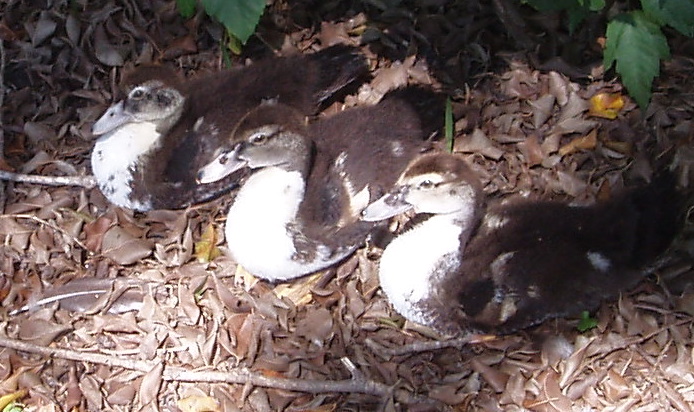In this daytime close-up photograph, three ducklings are nestled side by side on a bed of dried brown leaves, with various brown sticks woven throughout and a few yellow leaves scattered across the ground. The ducklings, sharing very similar markings, have fuzzy black heads and backs contrasted with white or off-white bellies and chests. Their small, dark eyes and gray beaks lend them a particularly endearing quality. Notably, the duckling closest to the camera on the right showcases a faint white patch on its face. All three ducklings are collectively gazing off to the left, intently focused on something beyond the frame. The backdrop features a dark green, vaguely triangular bush, adding depth and a touch of vibrant color against the otherwise earthy tones of the scene. While the image is a bit blurry, likely due to the close-up shot, it captures the tranquil moment in nature with a hint of charm.